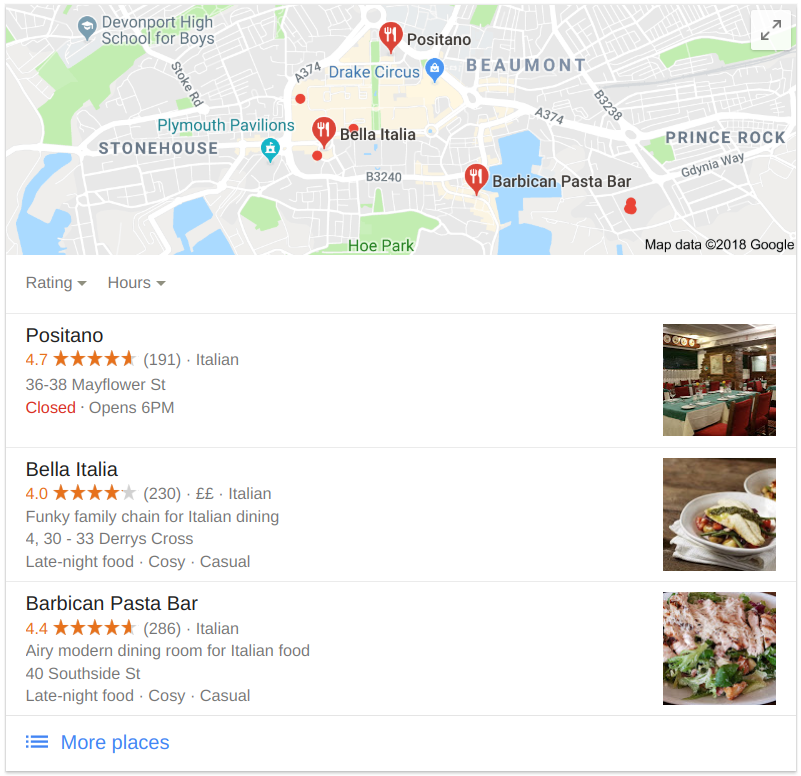At the top of the page, there's a map adorned with various location labels such as Devonport High School for Boys, Plymouth Pavilions, Stonehouse, Prince Rock, and Beaumont. The map, however, omits the name of the city but features three distinct red pins, each marked with a white fork and knife icon. 

The first pin, located centrally on the map, aligns with the text labeling "Bella Italia." The topmost pin is positioned near the label "Positano," while the pin furthest to the right is situated next to "Barbican Pasta Bar." The map also includes a note attributing the map data to Google in 2018.

Beneath the map, there is a detailed list of three restaurants:

1. **Positano**
   - **Rating:** 4.7 stars
   - **Cuisine:** Italian
   - **Address:** 3638 Mayflower Street
   - **Status:** Closed, Opens at 6 p.m.
   - **Image:** A photograph depicts the restaurant's interior, showcasing a table set with a tablecloth and chairs neatly arranged around it.

2. **Bella Italia**
   - **Rating:** 4.0 stars
   - **Cuisine:** Italian
   - **Description:** Funky family chain for Italian dining
   - **Additional Features:** Late Night Food, Cozy Casual
   - **Image:** To the right of the description, there is a photo displaying a bowl of food.

3. **Barbican Pasta Bar**
   - **Description:** Airy modern dining room for Italian food
   - **Additional Features:** Late Night Food, Cozy Casual
   - **Image:** Located to the right of the description, a close-up photograph highlights a plate of food.

The presentation offers a clear visual and textual guide, assisting in the selection of dining options based on preferences for cuisine, ambiance, and additional features.